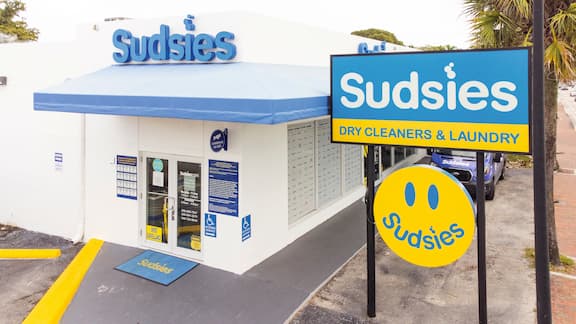This detailed daytime photograph captures the exterior of "Sudsy's Dry Cleaning and Laundry," showcasing a small white building with a blue awning. Prominently, there's a multi-part sign on black poles near the sidewalk. The top of the sign features a blue box with white letters spelling "Sudsy's" with the notable detail of the 'i' having three dots resembling soap bubbles. Below it, a yellow rectangle with blue text reads "Dry Cleaners and Laundry." Beneath this, a circular yellow sign includes a smiley face with eyes formed by blue ovals and the word "Sudsy's" making up the smile. The building itself is also adorned with similar signage and features a visible entrance. The environment includes a nearby road, a truck parked behind the sign, and several palm trees scattered around, giving a bright and welcoming tropical feel. The color palette consists predominantly of blue, yellow, white, greenish-yellow, green, black, and gray, enhancing the overall cheerful and clean aesthetic of the scene.